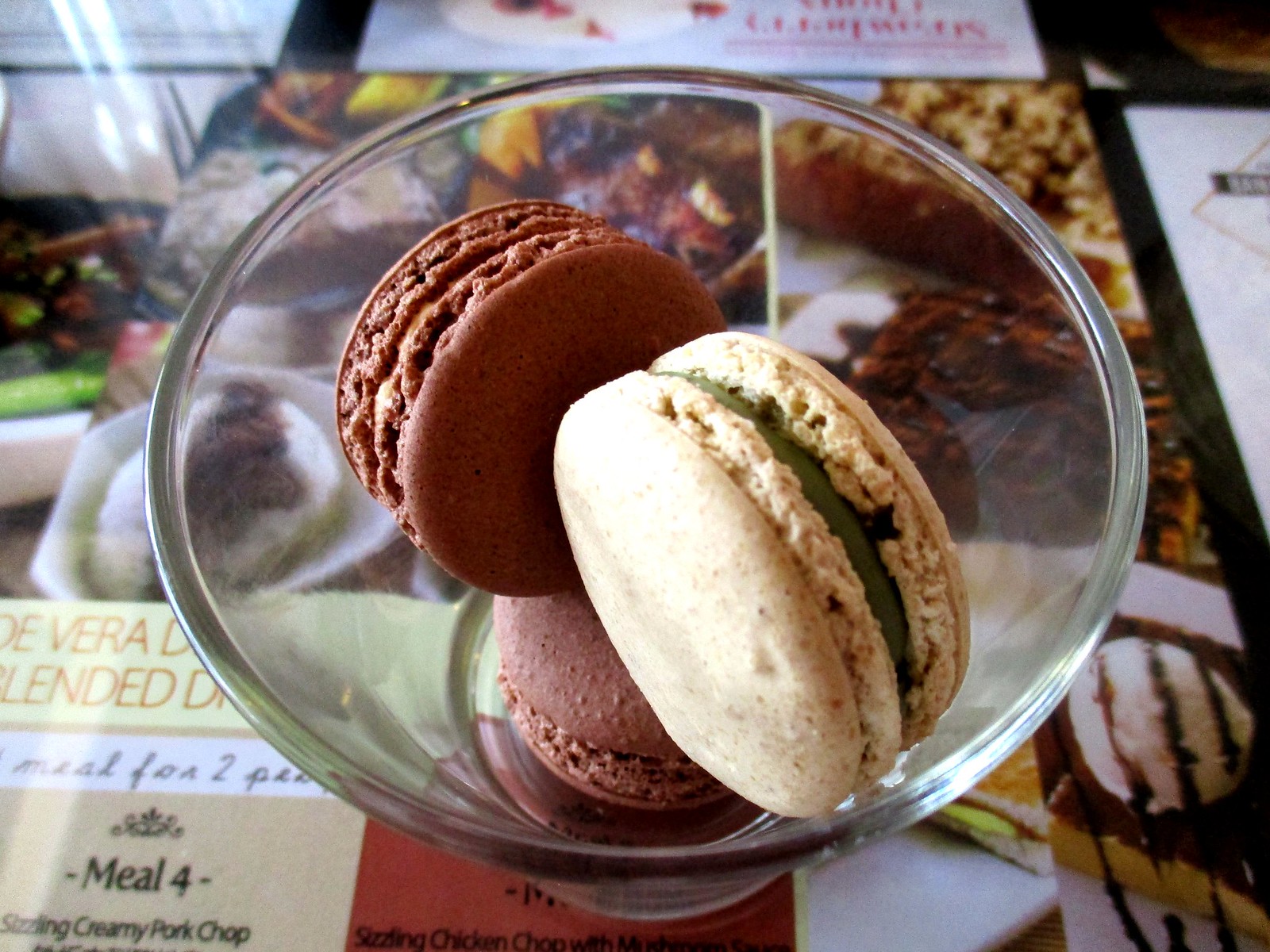In this close-up image, a clear glass container holds three macarons, displayed on a table with a laminated menu visible in the background. The macarons are arranged with one chocolate macaron, filled with chocolate, at the bottom, and two standing upright on top—one chocolate with chocolate filling, and one off-white or vanilla with a green filling, possibly pistachio. The table's menu board, though partially obscured and out of focus, features various food items, including sushi, vegetables, and desserts like ice cream with chocolate syrup. Visible text on the menu reads "D'Vera D, blended D, meal for two," and "sizzling creamy pork chop." This vibrant scene suggests a restaurant setting with a diverse menu.